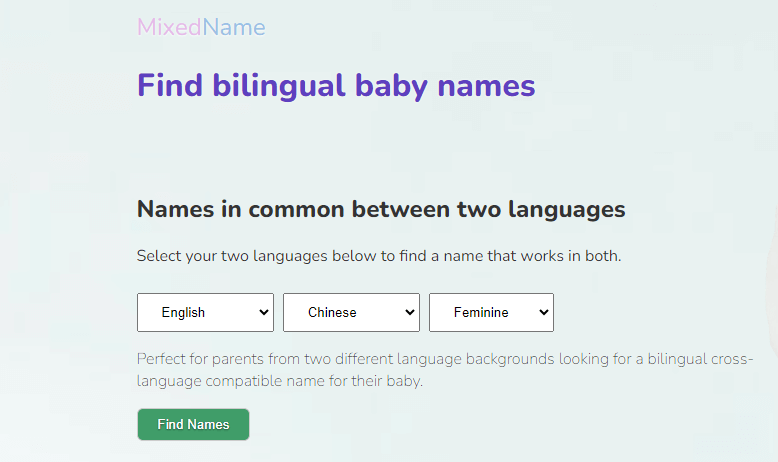Looking for the perfect bilingual baby name that works seamlessly in both English and Chinese? Explore a curated selection of feminine names that are common to both languages, ideal for parents from diverse cultural backgrounds. Choose names that carry meaning and charm in both English and Chinese, ensuring a beautiful cross-language compatibility for your little one.